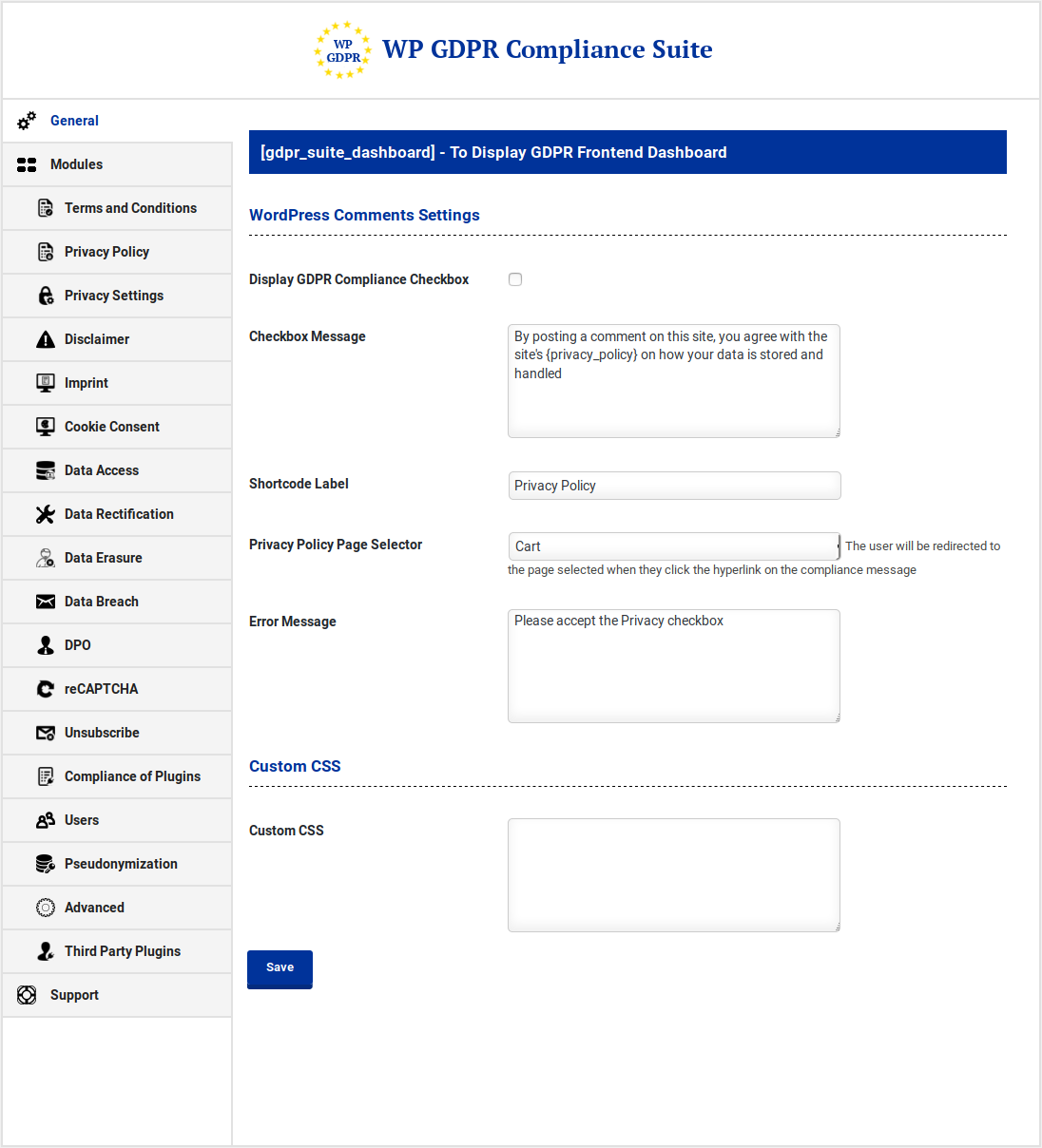**Detailed Caption for the Screenshot:**

At the top center of the screenshot, "WPGDPR Compliance Suite" is prominently displayed in blue lettering. Along the left-hand side is a vertical list of menu options, each button shaded gray with black text, except for "General," which is highlighted in the same blue color as the title. The menu begins with "General" and continues with "Modules," "Terms and Conditions," "Privacy Policy," "Privacy Settings," "Disclaimer," "Imprint," "Cookie Consent," "Data Access," "Data Rectification," "Data Erasure," "Data Breach," "DPO," "ReCAPTCHA," "Unsubscribe," "Compliance of Plugins Users," "Sued Anonymization," "Advanced," "Three-Party Plugins," and "Support."

Beneath the main title, there is a blue banner that reads "[GDPR__Suite__Dashboard] GDPR Front End Dashboard" followed by "WordPress." Below this, there are several settings options: "Comment Settings" with "Display GDPR Compliance Checkbox," followed by "Checkbox Message" next to an input box, then "Shortcode Label" beside another input box. The "Privacy Policy" section follows, which includes "Privacy Policy Page Selector," "CART," and an adjacent larger input box for "Error Message." 

At the bottom, there is a section labeled "Custom CSS," with an input box next to it, and a blue "Save" button below this input area. The screenshot captures the detailed layout of the GDPR compliance configuration settings within a WordPress environment.